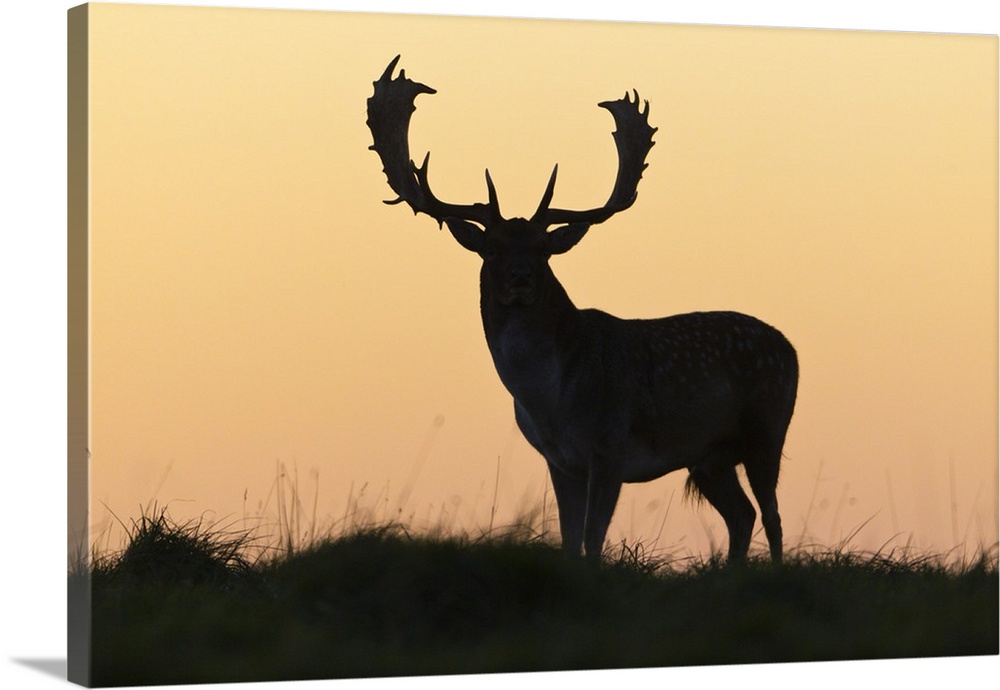A captivating piece of outdoor art, this full-color photograph is ready to hang and appears tilted diagonally to the right. Set in a square frame that casts a shadow at the bottom, the image showcases a majestic deer, possibly a buck, with an impressive set of antlers featuring sharp points in the center and prongs that resemble sticks. The deer, depicted in black silhouette or faint shadow, stands amidst high grass or tall weeds in the foreground. The background is bathed in a rich orange-yellow glow of the sky, suggesting the time is either early evening or early morning, just as the sun is setting or rising. The scene is vivid yet subtle, capturing a moment of natural beauty and tranquility.